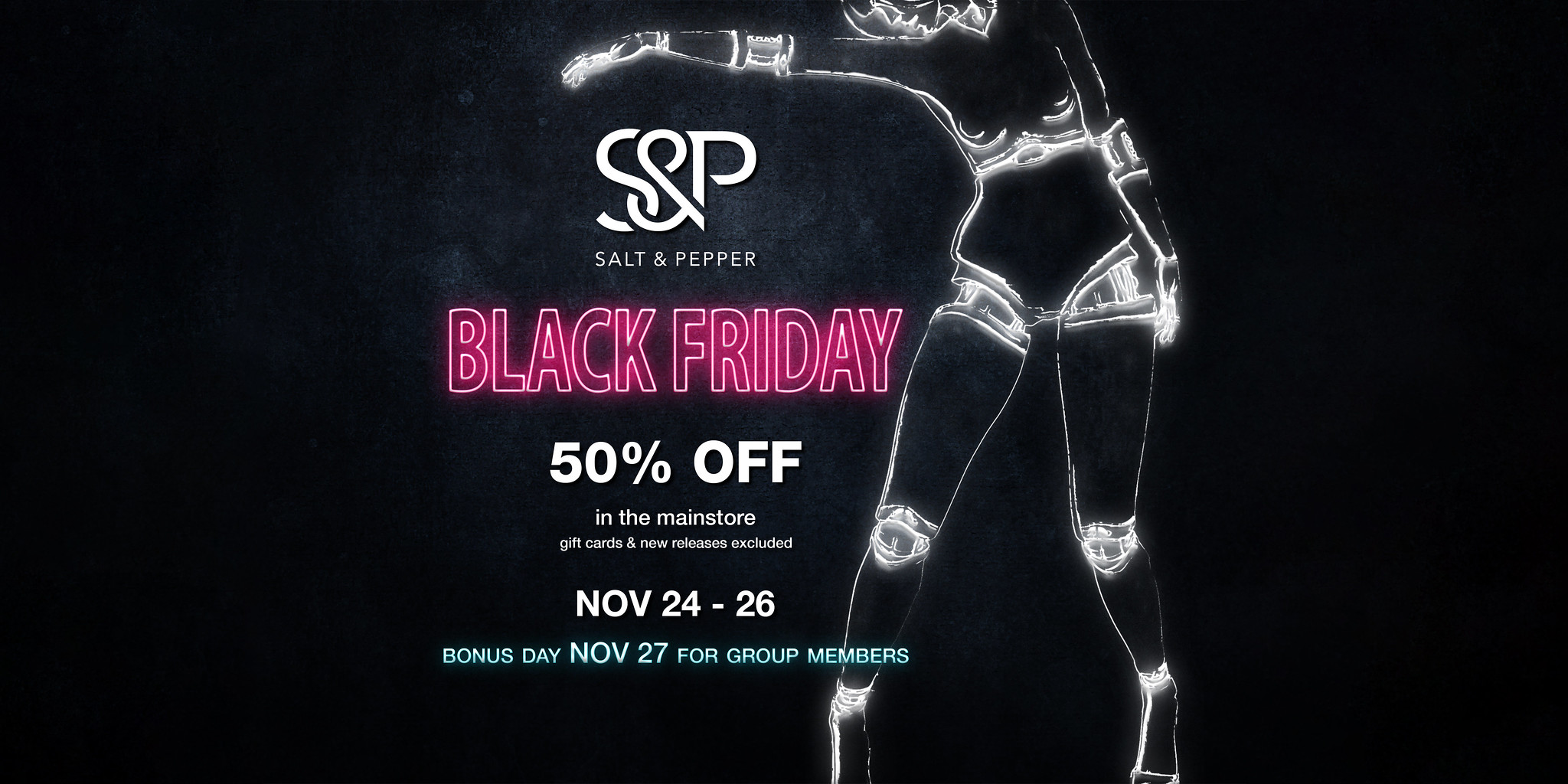The advertisement features a striking digital illustration set against a black background, creating a futuristic and cyberpunk aesthetic. Central to the image is the translucent silhouette of a thin woman rendered in white neon outlines, highlighting her joints including her hips, elbows, wrists, and ankles, while the inside of her body remains black. She is adorned in athletic attire comprising a jersey, shorts, knee pads, and shoes. Her right arm extends across the top of the image, under which the white letters "S&P" and the text "Salt and Pepper" appear. In large neon pink letters, it reads "Black Friday," followed by white text that announces "50% off in the main store," with a note that gift cards and new releases are excluded. The dates for the sale are November 24th through 26th, followed by a smaller blue text indicating a "Bonus Day" on November 27th for group members.